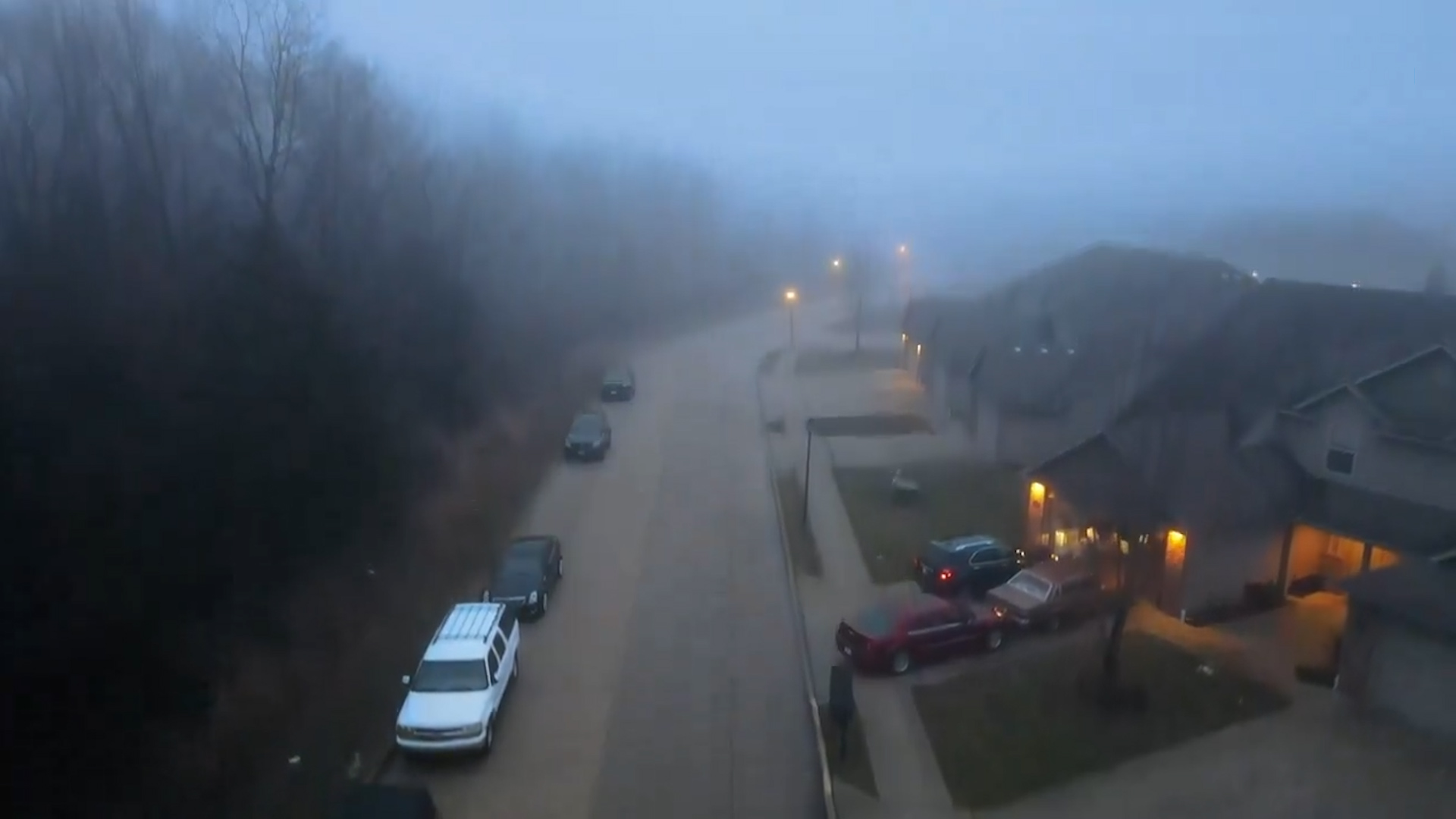The image depicts an overcast, foggy suburban street scene captured from an elevated angle, possibly a street camera or drone. The atmosphere suggests it is either at dusk or dawn, with limited visibility due to the fog. On the left-hand side, a dense, leafless wooded area extends upward, indicating it's winter. In front of the trees, five vehicles are parked on the street, including four dark-colored cars and one white SUV. The street runs down the center of the image, veering slightly to the right as it recedes into the fog-covered distance.

On the right-hand side, two fully visible houses stand out with their front porch and task lights turned on. These homes, painted in neutral tones like gray, brown, or tan with gabled roofs, have small front yards. The foreground house's driveway is occupied by three cars: a red car, a black SUV, and an older brown sedan, with at least two of them showing illuminated taillights. Overall, the ambient scene is hushed, empty of human activity, and also features several street lights faintly visible in the distance through the fog.